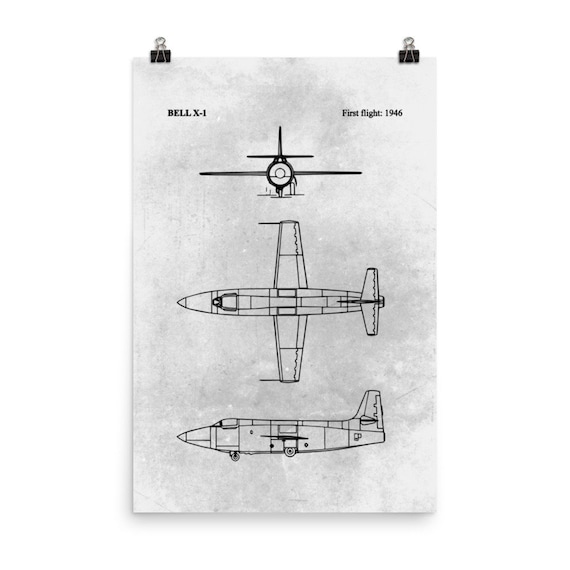The image showcases a detailed black and white drawing of the Bell X-1 jet, accompanied by the text "First Flight, 1946" at the top. The drawing features three different perspectives of the airplane: a head-on view from the front, highlighting its circular nose, main wings, smaller tail wings, and fin; a top-down view, displaying the aircraft's full design from above; and a side view, revealing the jet's pointed nose, tail fin, and set of wheels. The drawing is held up by two black and silver binder clips against a white background, with the paper itself being a slightly darker shade. The overall sketch is very detailed yet simplistic, accurately presenting the Bell X-1 from multiple angles without any color, relying solely on shades of white and black for representation.